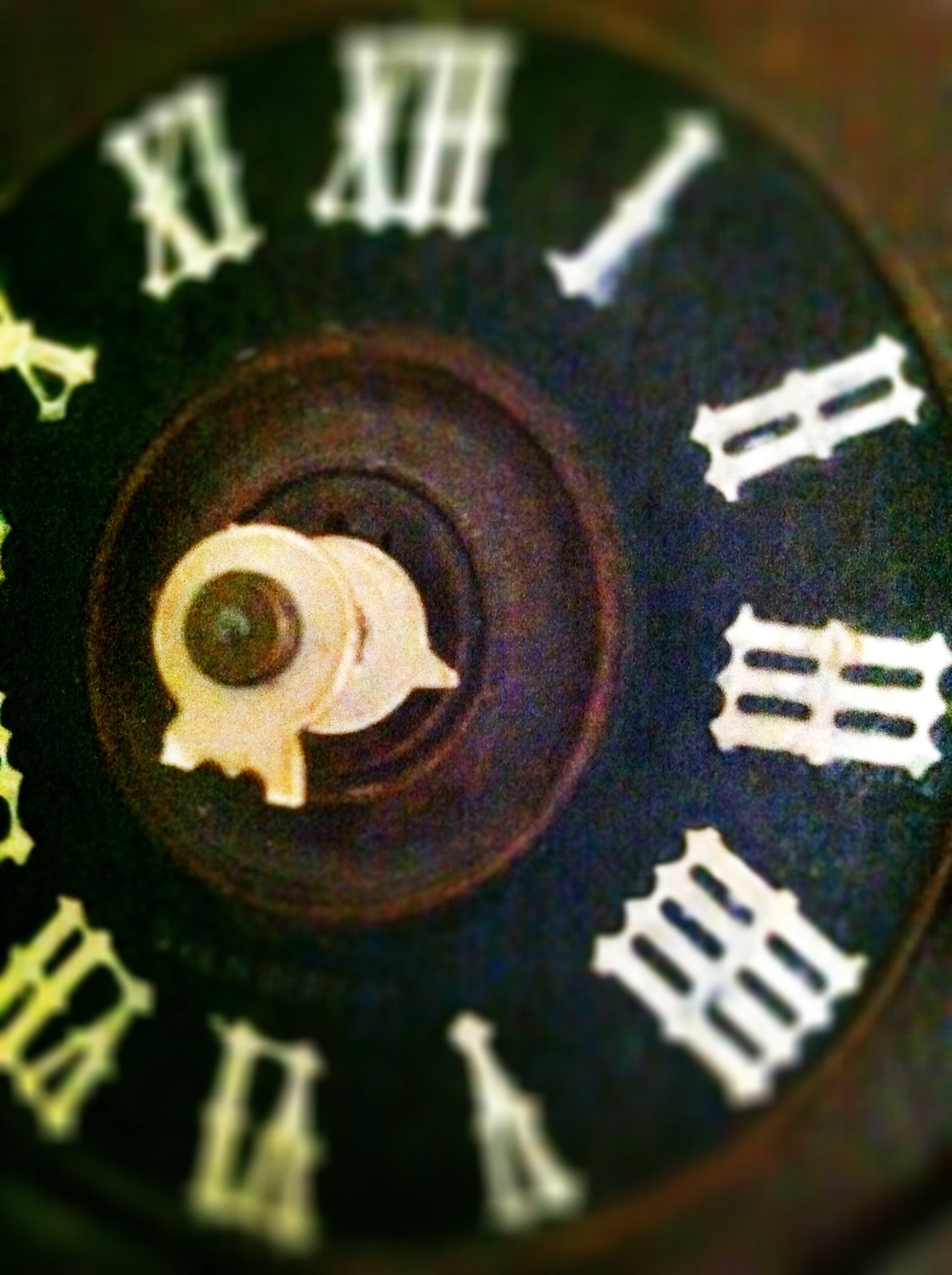This close-up photograph showcases a weathered and antiquated clock that appears to be broken. The image prominently features the clock's center, where the hands once connected; however, the hands are now missing, leaving behind a small white portion and a protruding remnant. Surrounding the central axis, there is a rusty, metallic ring that adds to the clock's aged appearance. The clock face itself is black and adorned with Roman numerals, though the focus on the numerals varies. The numbers II, III, and IV on the right side are clear, while the remaining numerals are smudged and blurred. The design of the Roman numerals is reminiscent of a white picket fence, with lines at the top, middle, and bottom for each digit, adding a unique visual element to the clock's overall dilapidated aesthetic.